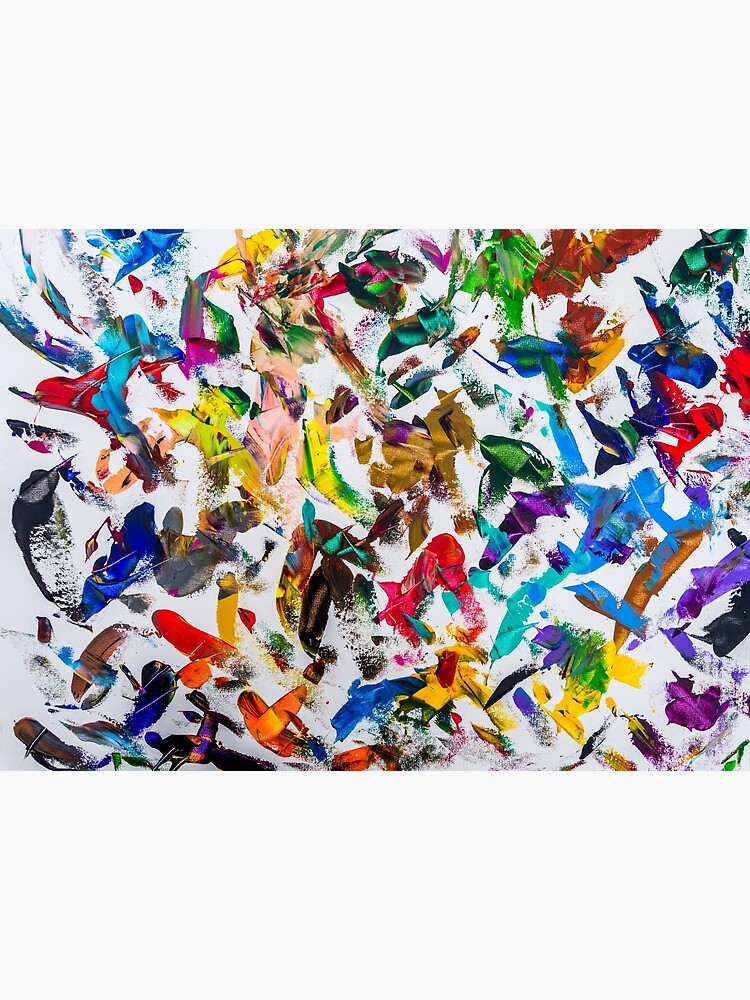This image showcases a vibrant and abstract painting bordered by white at the top and bottom. The central focus is a riotous and colorful collage of paint swatches on a white canvas, featuring a plethora of hues including reds, blues, yellows, purples, oranges, pinks, greens, browns, and blacks. The daubs and smears of various colors are arranged in seemingly random, overlapping patterns, with no discernible figures or text. The absence of any recognizable shapes or artist attribution underlines its modern and abstract nature. The composition emphasizes a lively and bright palette, predominantly using primary colors over pastels, reflecting a dynamic, non-representational design.